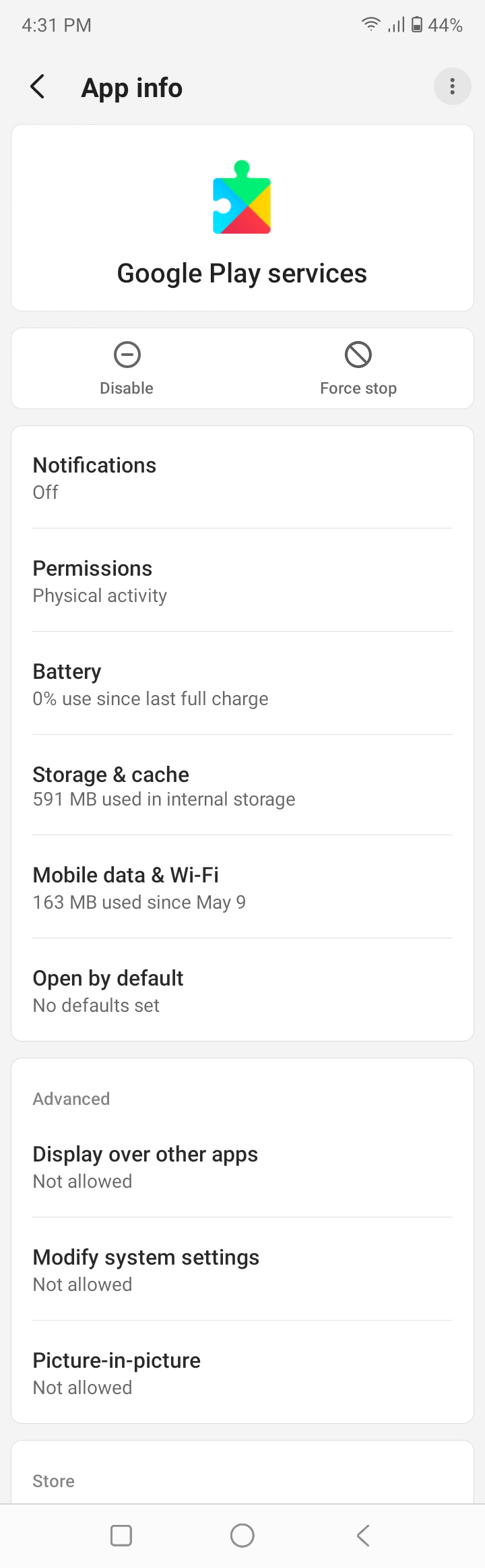The image depicts the "App Info" screen of a smartphone displaying details for Google Play Services. The time displayed in the status bar at the top left is 4:31 PM, accompanied by icons indicating Wi-Fi signal strength, cellular reception, and a battery level of 44%.

At the top of the "App Info" screen, there is a back arrow on the left side and three vertically aligned black dots within a gray circle on the right side, indicating additional options. Directly below, a white rectangular area features the Google Play Services icon, a multicolored puzzle piece in green, blue, orange, and red, alongside the app's name "Google Play services."

Beneath this area are two side-by-side buttons: "Disable," marked with a gray circle and a line through it, and "Force stop," indicated with a gray circle and a diagonal line through it.

The next section details various parameters in a list format:
- **Notifications**: Manage notifications for the app.
- **Offline Permissions**: Permissions related to offline activities.
- **Physical Activity**: Permission to access physical activity data.
- **Battery**: "0% usage since last full charge."
- **Storage & Cache**: "591 MB used in internal storage."
- **Mobile Data & Wi-Fi**: "163 MB used since May 9th."
- **Open by Default**: "No defaults set."

Following this is another rectangular area labeled "Advanced," containing additional settings:
- **Display over other apps**: "Not allowed."
- **Modify system settings**: "Not allowed."
- **Picture-in-picture**: "Not allowed."

Below this advanced settings rectangle is a partially visible section titled "Store," though the text is cut off.

At the bottom of the screen, the phone's navigation bar is visible, displaying the standard icons for "Back" (a backward arrow), "Home" (a circle), and "Recent Apps" (a square).